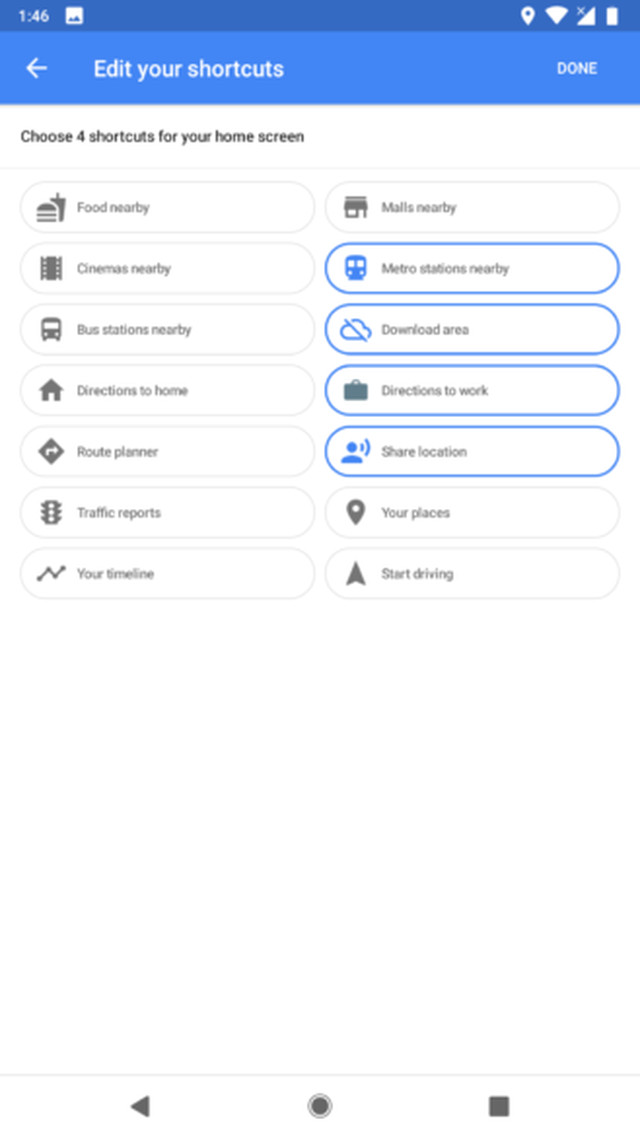At the top of the image is a dark blue rectangle. Directly beneath it, there is a thicker, light blue rectangle with a left-pointing arrow in its center. The light blue rectangle features the words "Edit your shortcuts" in white text, followed by the word "Done." 

Below this light blue section, a white background displays a black text header that reads, "Choose four shortcuts for your home screen."

Underneath this header, the image is divided into two columns of text. The left column contains multiple entries:
1. Food Nearby
2. Something Else Nearby (text is very small and hard to read)
3. Something Else Nearby
4. Bus Stations Nearby
5. Something to Home
6. Route Planner
7. Traffic Reports
8. Your Something (again, unclear text)

The right column lists:
1. Malls Nearby
2. Something Else Nearby
3. Download Area (outlined in blue with an icon in front)
4. Directions to Work (outlined in blue with an icon in front)
5. Share Location
6. Your Places
7. Start Driving

The entries "Download Area," "Directions to Work," "Share Location," and "Start Driving" are particularly highlighted with a blue outline and include small icons adjacent to the text.